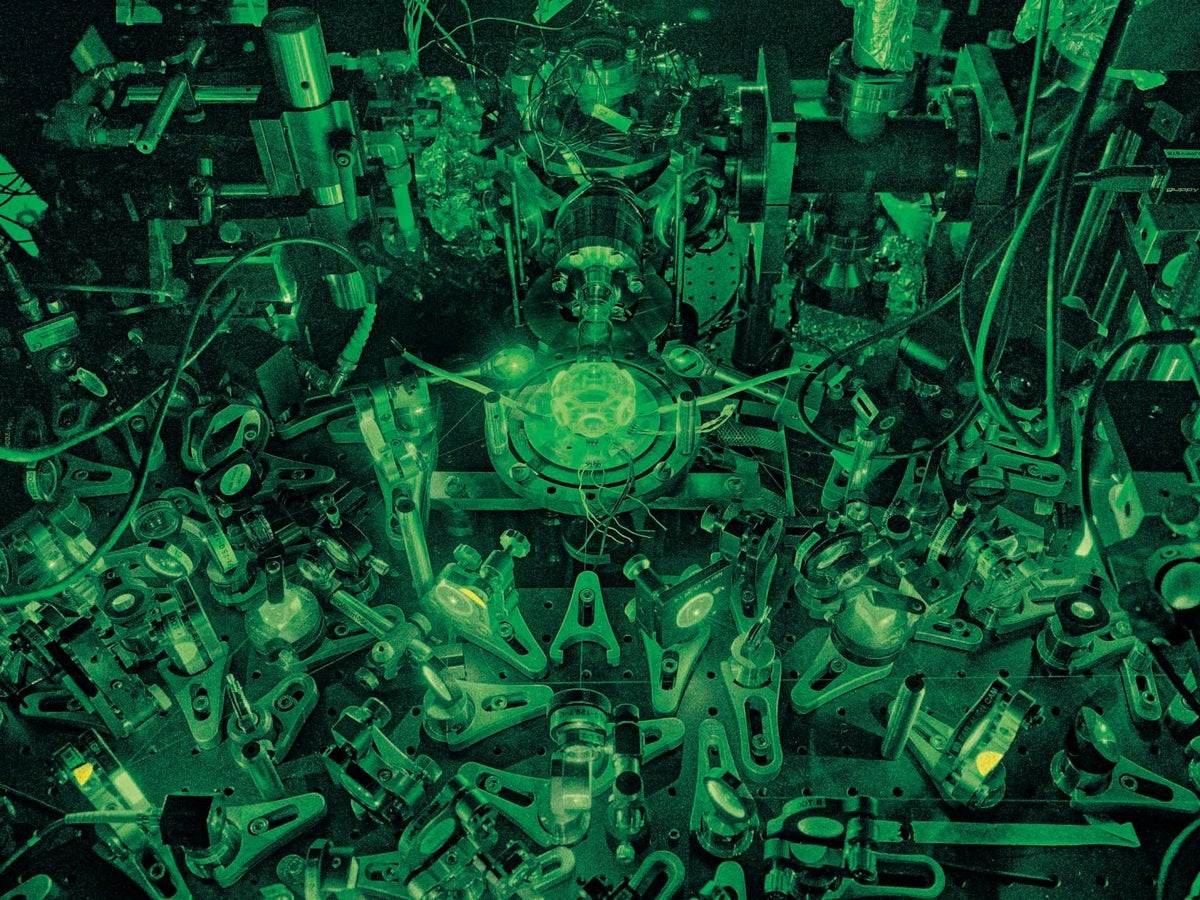The image displays the intricate inner workings of what appears to be a mechanical or computer device, bathed entirely in a green tint, possibly due to specific lighting rather than the components' actual colors. Dominating the center is a circular plate, highlighted and surrounded by small round circles. This plate is interconnected by numerous wires extending to various parts of the device. Clamps or clips, some in a V-shape with holes set on protruding rods, are scattered around, particularly through the bottom middle section. The background, contrasting in black, hosts vertically and horizontally oriented elements, including cylindrical objects that resemble capacitors. The entire setup suggests a complex scientific experiment or a highly detailed component of a computer or mechanical system.